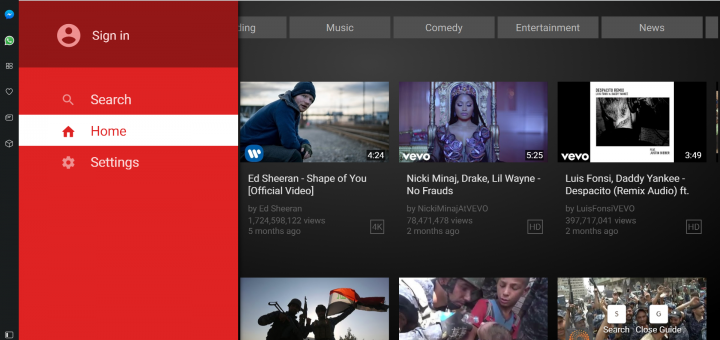The image displays a detailed layout of a web page. On the left side of the page, there is a navigation menu that includes options such as Messenger, WhatsApp, Sign-in, Search, Home, and Settings. The main content of the page features several music videos.

At the top, there is a video of Ed Sheeran's "Shape of You (Offshore Video)" which has garnered 1,724,598,122 views and was uploaded 5 months ago. It is available in 4K resolution. Below it is a music video titled "No Frauds" by Nicki Minaj featuring Drake and Lil Wayne, boasting 78,471,478 views. Following this, there is an audio-only remix of "Despacito" by Fonzie and Daddy Yankee, with 397,717,041 views and posted two months ago. 

The bottom section of the page shows additional videos that lack captions. The color scheme of the page prominently features red, white, green, blue, and black.